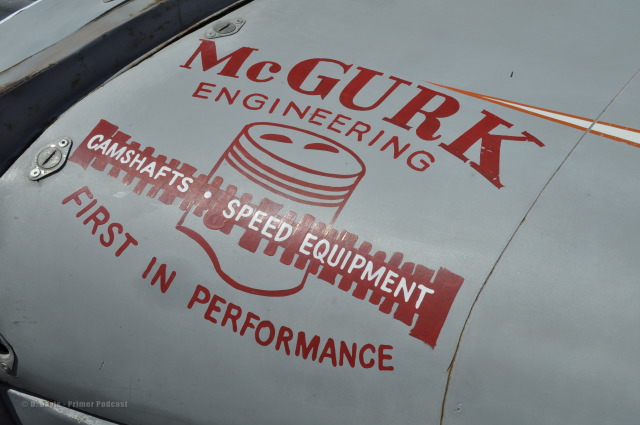This image features a close-up shot of what appears to be the trunk of a car, characterized by a curved sheet metal surface in a shade of gray. Dominating the center of the image is a distinct logo in red lettering that reads "McGurk" with a small 'c' and capitalized "GURK" alongside the word "ENGINEERING" all in uppercase. Beneath the logo, there's an eye-catching red background banner with white text that says "CAMSHAFTS • SPEED EQUIPMENT." Overlaying this is a graphic depiction of a camshaft, rendered in red, featuring cylindrical shapes with bands and markings. Below this graphic, the text "FIRST IN PERFORMANCE" is prominently displayed in all caps. Additional elements in the photo include large screws visible off to the left side, adding to the mechanical essence of the image. The predominant colors in this detailed composition include gray, red, white, silver, and black, emphasizing the engineered and industrial nature of the subject.